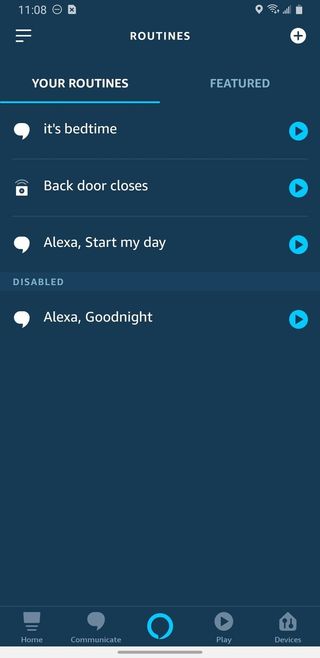The image is a screenshot from a mobile app. At the top center of the screen, there is a header labeled "Routines." To the left of this label is a three-line menu button, and to the right is a white circle containing a blue plus sign.

Below the header, there are two tabs. The first tab, which is selected, is labeled "Your Routines." Under this tab, the app lists various routines including "Bedtime," "Back Door Closes," and "Alexa, Start My Day." There is a separation that indicates disabled routines, under which it reads "Alexa, Good Night." 

To the right of the "Your Routines" tab is another tab labeled "Featured," although it is not selected in this screenshot. 

The background of the app is dark blue, and there is a notable portion of blank space before reaching the bottom navigation bar. 

The bottom navigation bar consists of five buttons. From left to right, they are "Home," "Communicate," a central Alexa button symbol, "Play," and "Devices." 

The time displayed on the screen is 11:08.